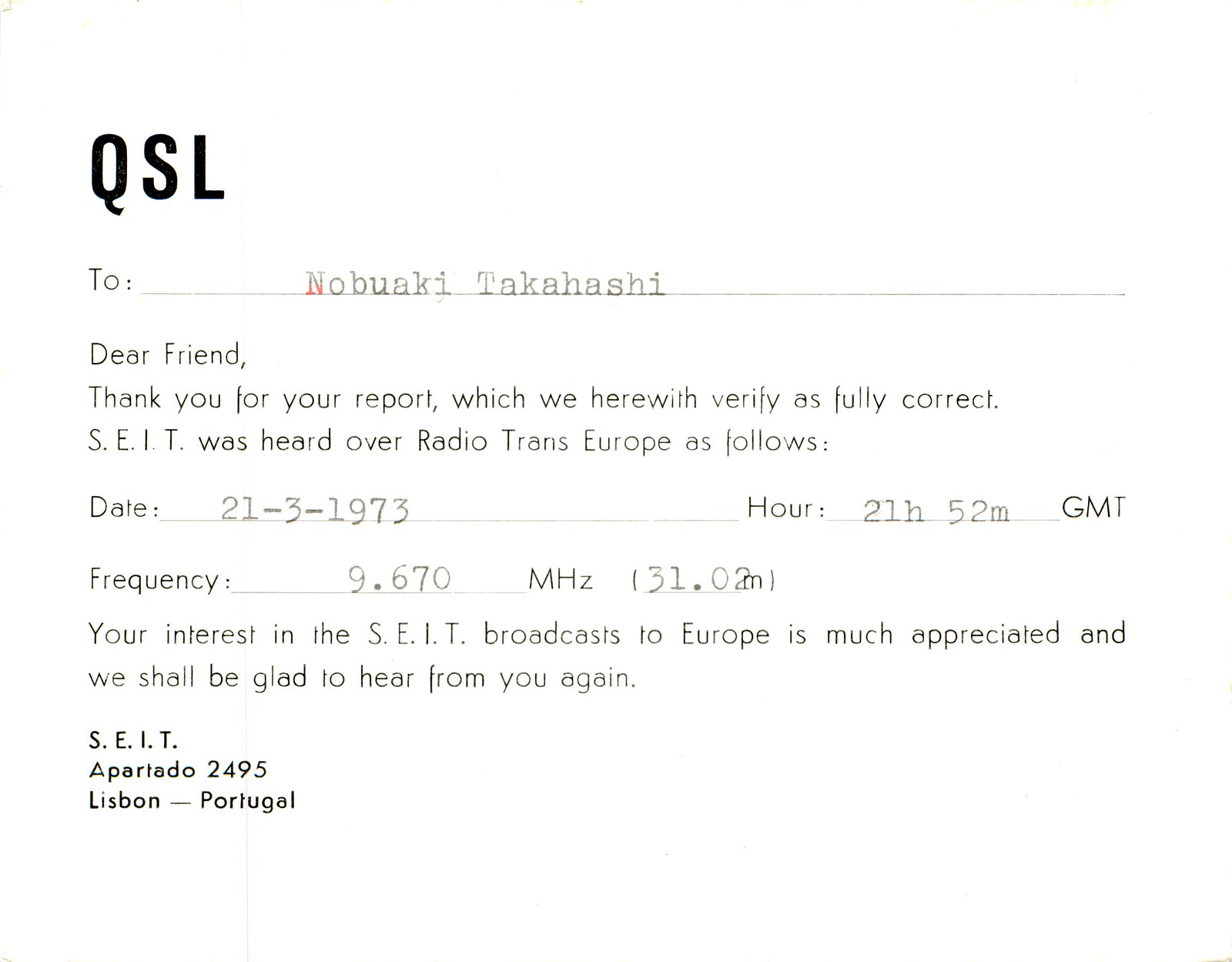This image depicts a black-and-white, landscape-oriented document on a white but slightly yellowed background, designed as a verification of a radio broadcast. The top left corner prominently displays the bold, condensed uppercase letters "QSL," followed underneath by "2:" and a long line with the typed name "Nobuaki Takahashi." Below, a pre-printed message reads, "Dear Friend, thank you for your report, which we herewith verify is fully correct. SEIT was heard over Radio Trans Europe as follows." The document records details of the broadcast, including the date "21-3-1973," the time "21H52M GMT," and the frequency "9.670 MHz" (31.02M). It continues, "Your interest in the SEIT broadcast to Europe is much appreciated, and we shall be glad to hear from you again." The lower left corner features the typed address: "SEIT, Apartado 2495, Lisbon, Portugal."